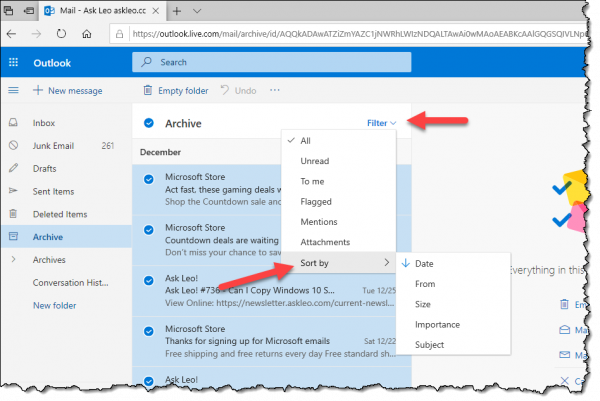The image showcases a Microsoft Edge browser window with Microsoft Outlook open. The interface prominently displays the "Archive" menu, under which five emails are archived. Highlighted within the interface are several options: the "Sort By" menu, marked with a red arrow, and the "Filter" menu, also indicated by a red arrow. The "Sort By" dropdown reveals choices such as Date, From, Size, Importance, and Subject, illustrating the functionalities available for organizing archived emails. The screenshot itself has a unique visual treatment, with rough, burnt-looking edges and a drop shadow effect, suggesting the image was selected and modified using a rough-edged brush tool.